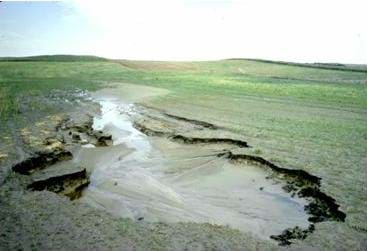This image depicts an outdoor scene with a blurry, low-resolution quality. The sky at the top of the image is a mix of bright white and blue, indicating either sunrise or strong sunlight. In the background, there are gently sloping green hills. The foreground features an expansive field with short, green grass. Prominently in the center of the image is a jagged-edged crevice or sinkhole filled with muddy water, surrounded by patches of dry, rocky terrain. The sun's brightness renders part of the image difficult to see, lending an almost washed-out appearance to the sky and casting light across the landscape. The greenery and natural elements dominate the scene, with the central water-filled feature drawing particular attention amidst the field.